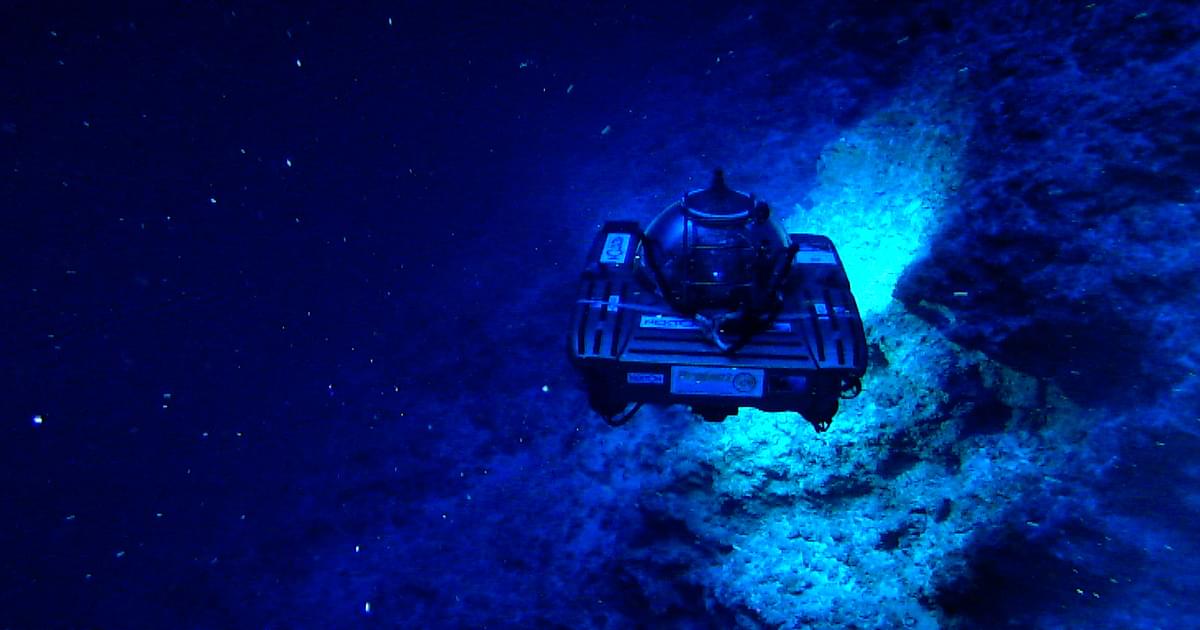The image portrays a dark, otherworldly scene dominated by shades of blue, suggesting a setting in space or underwater. The sky—or possibly water—on the left side is a deep, almost navy blue, speckled with variously sized white dots that resemble stars. Central to the image is a vessel that brings to mind both a tank and a spaceship, featuring a turret-like, rounded cockpit akin to a robotic or drone head. The vessel, tinted in royal blue, is complemented by fender-like wings extending forward from its main body and detailed with black horizontal stripes.

To the right side of the vessel, a formation resembling a shelf of blue lava rocks or underwater rocks is illuminated by a bright aqua light. This vivid illumination also highlights parts of the cloud-like formations around it. Further detailing reveals that the vessel has pipes attached below it, contributing to the intricate design of its structure. The overall scene is reminiscent of a video game or a computer-generated image, with its detailed textures and the interplay of light and shadow, creating a rich, atmospheric depiction.